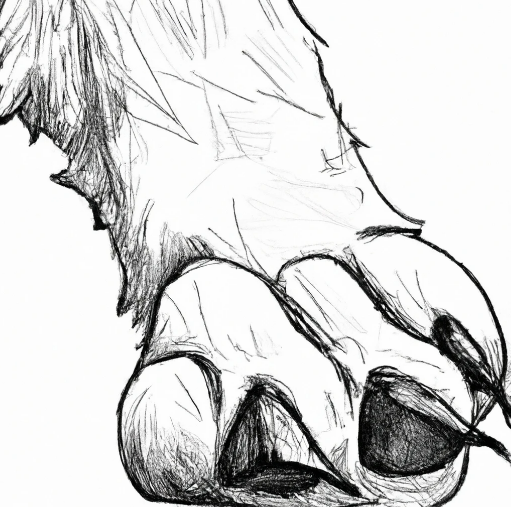This image features a black-and-white illustration of an unidentified animal's paw. The paw, drawn with a fine attention to detail, is depicted with three rounded toes that feature prominent, sharp, black claws. The entirety of the toes is accentuated with scratchy, white lines, showcasing the artist's intricate shading work. Extending from the toes, the lower part of the leg, or shin, displays jagged fur outlines transitioning into smoother lines towards the toes. The leg is rendered in white, interspersed with varied, shaded black lines, giving a textured and nuanced appearance to the fur. Spanning diagonally across the square image, the paw and leg contrast starkly against the pure white background, enhancing the visual impact. Overall, the illustration adeptly captures the light coming from the upper right corner, casting deep shadows that emphasize the form and texture of the paw and its menacing claws.